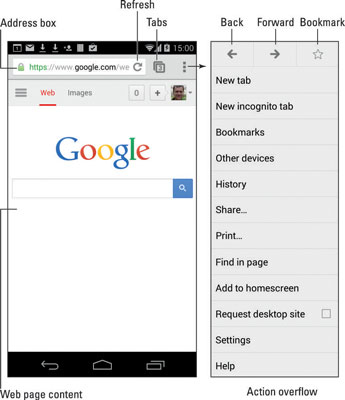A detailed caption for the described images could be:

"The composite image showcases two side-by-side screenshots. The left screenshot appears to be from an antiquated version of Android, displaying Google's homepage. At the very top, a black status bar indicates the time as 15:00, along with battery, Wi-Fi, and cell signal icons, as well as notifications aligned on the left. The bottom of the screenshot features old Android icons for navigation. Prominently, the Google homepage is centered, featuring the Google logo in its colorful design and a large search bar beneath it. At the top right corner, both a hamburger menu (three horizontal lines) and a three-dot menu button are visible. An arrow extends from the three-dot menu button into a white space, leading to the right screenshot.

The right screenshot captures the dropdown menu that appears when the three-dot button is pressed in the Google Chrome browser. Listed menu items include New Tab, New Incognito Tab, Bookmarks, Other Devices, History, Share, Print, Find in Page, Add to Home Screen, and more. The layout is annotated with black lines connecting to various elements: one pointing to the address box with a label 'address box' and another pointing to the refresh button with the label 'refresh'."